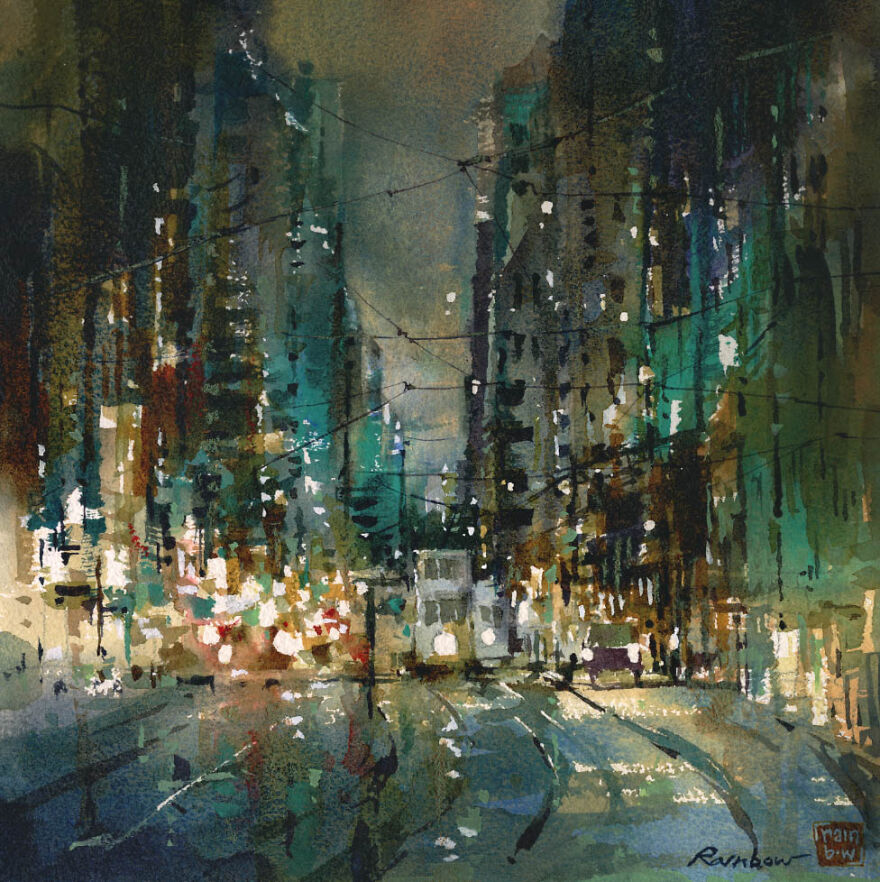This image is a photograph of a watercolor painting titled "Wilshire Boulevard at Night" by the artist Emil. The painting, which has a square format, depicts a nocturnal cityscape brimming with intricate details and muted yet dynamic colors. The scene centers on a curved city street that draws the viewer’s eye towards an array of towering skyscrapers and buildings, rendered in swashes of dark blue, brick red, and gray. The composition is bisected by a bustling thoroughfare, populated with boxy-shaped vehicles, including a prominent trolley car on the tracks and another smaller one beside it. Overhead, strings of lights cross the street, enhancing the atmospheric depth of the scene. The color palette features shades of blue, green, and brown with a touch of red, all contributing to the painting’s abstract, impressionistic quality. The artist's signature, "Rainbow," is inscribed on the bottom right corner, next to a distinctive red box also labeled "Rainbow." This evocative painting captures the vibrancy of city life with a unique blend of abstraction and realism.